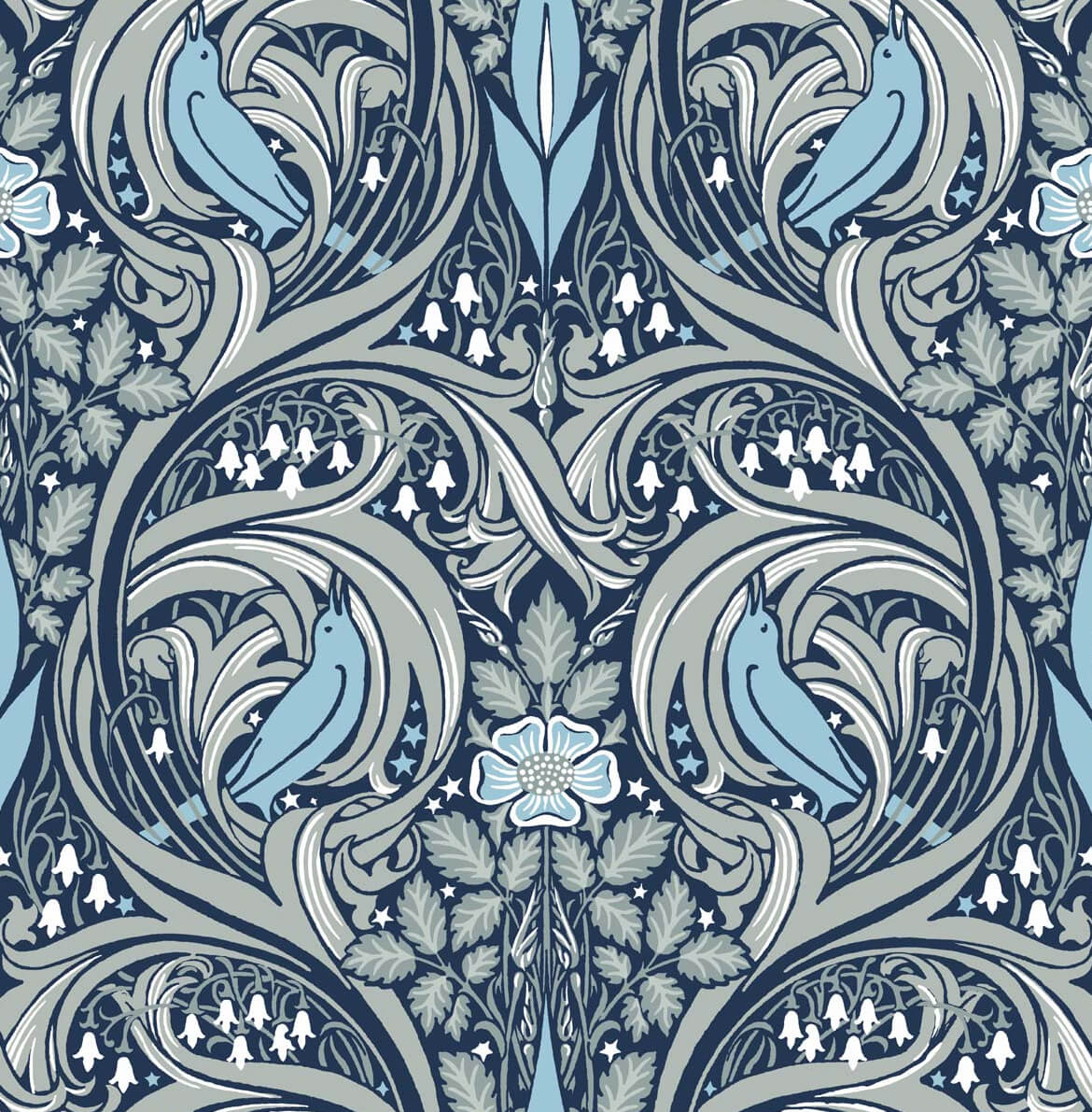This intricate and repeating pattern resembles an elegant wallpaper, featuring a harmonious blend of gray, dark blue, light blue, turquoise, and white. At the heart of the design, a prominent flower is surrounded by stylized elements, including various buds and leaves. The motif highlights eight birds, all depicted in a light blue hue, with subtle white streaks adding depth and detail. 

The birds are symmetrically arranged: two are facing away from each other at the top, while two at the bottom face towards one another. On either side of the central flower, there are matching pairs of birds facing opposite directions. The birds exhibit delicate features like beaks, outlined wings, and eyes, enhancing the intricate aesthetic of the artwork.

The overall composition contains numerous floral elements, including flowers with white pollen centers, leaves, and swirling ribbon-like patterns that evoke a paisley style. The repeated nature of the design makes it well-suited for use as wallpaper or fabric, adding a touch of sophistication and tranquility to a room with its beautiful, artistic arrangement of blues and grays.